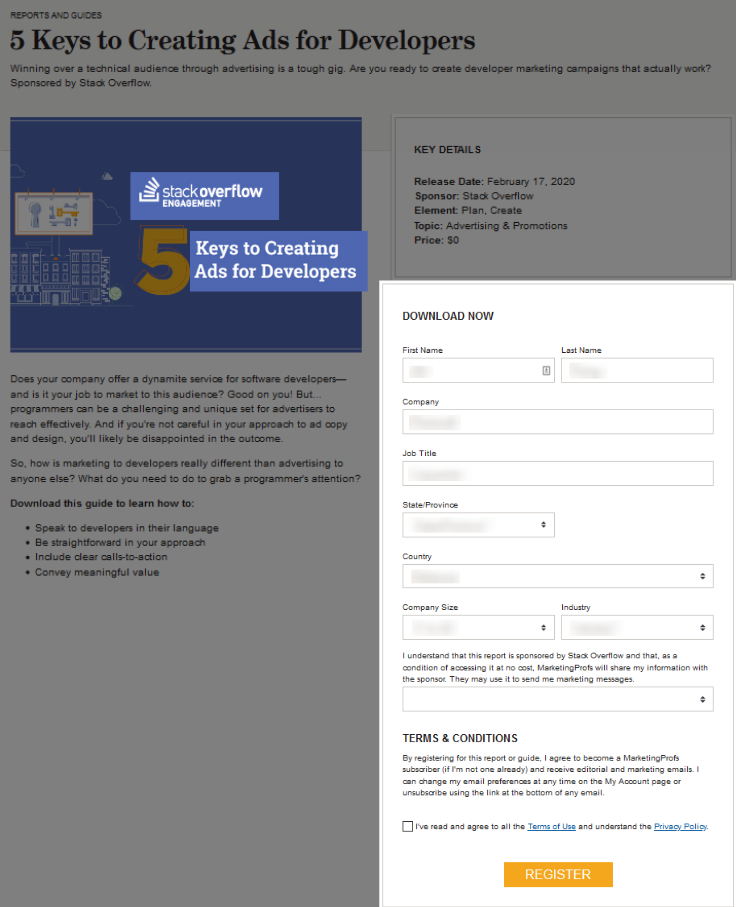Sure, here's a detailed caption for the image described:

"This color, portrait-format screenshot captures a webpage featuring an article aimed at marketers focused on creating advertising for software developers. The article titled 'Five Keys to Creating Ads for Developers' is prominently displayed, highlighting the challenge of engaging a technical audience. The section reads: 'Winning over a technical audience through advertising is a tough gig. Are you ready to create developer marketing campaigns that actually work?' This guide, sponsored by Stack Overflow, offers insights on effective developer marketing strategies, emphasizing the need for succinct, clear, and value-driven approaches to appeal to programmers. The page urges companies providing services to software developers to download the guide for advice on crafting ads that resonate with this unique audience. A registration form at the bottom-right corner prompts users to enter personal and professional details, such as first name, last name, company, job title, state, country, company size, and industry. The form concludes with an option to accept terms and conditions in order to download the guide."

This caption provides a comprehensive description of the image's content and context.